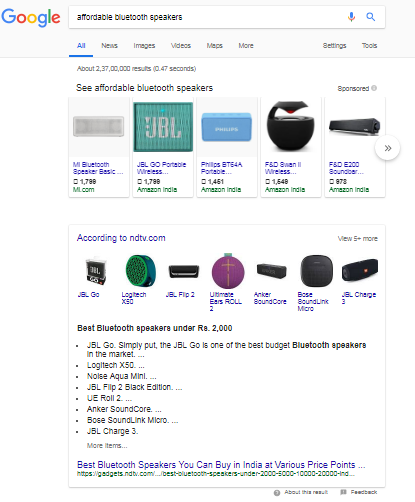A vertical image showcases a Google search page, captured either from a computer or a smartphone. At the top, the iconic Google logo appears in its traditional colors (blue, red, yellow, blue, green, red) against a gray background. Below the logo, the familiar white search bar is present, complete with a microphone icon and a magnifying glass icon on the right side.

The search query entered is "affordable Bluetooth speakers." Beneath the search bar, navigation options are displayed, including "All," "News," "Images," "Videos," "Maps," and "More," with "All" highlighted in blue. To the right, there are options for "Settings" and "Tools."

The search results indicate the number of results and the time it took to generate them. The results include images of various Bluetooth speakers, with their names and prices listed underneath. Some results are marked as sponsored ads. 

Further down, a section attributed to NDTV.com appears, listing affordable Bluetooth speakers with a series of bullet points detailing features and specifications for items priced under 2000.